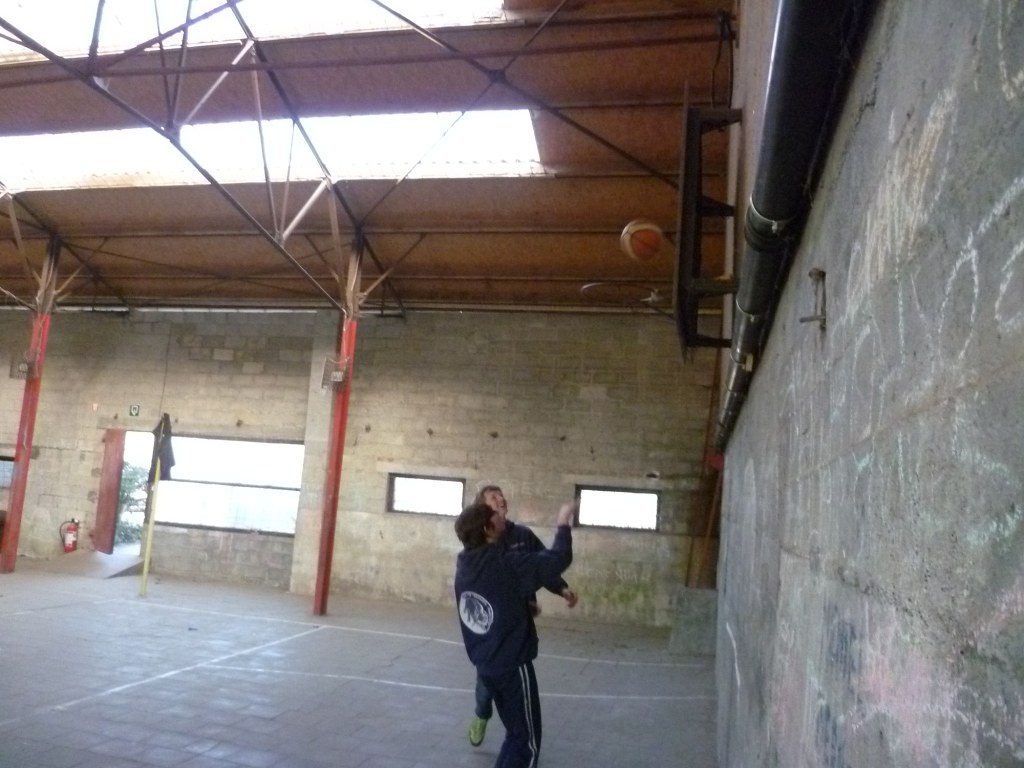In this image, two men are seen shooting a basketball inside an unfinished indoor gym that looks like a mix between a basement and a warehouse. The surroundings include gray concrete floors with white painted lines and cinder block walls adorned with chalk writings. The gym is further characterized by exposed metal scaffolding and support poles, with the ceiling featuring large skylights and several windows that allow ample natural light to flood the space. The basketball hoop is visible above, though it appears without a net, and there's a backboard that isn't fully visible due to the side angle of the shot. The men are dressed in black track suits with white stripes, and one of them has an indistinct white logo on the back of his attire. Despite the rough, industrial surroundings, they are clearly engrossed in playing basketball and enjoying their time.